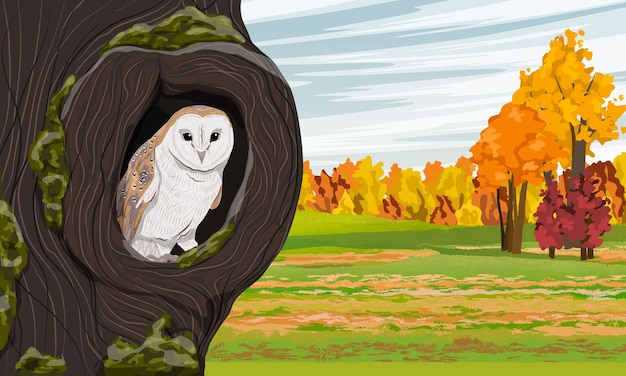This detailed illustration, resembling a digital or watercolor painting, captures an intimate outdoor scene on an overcast fall day. The sky is painted with wispy, grayish-white clouds, enhancing the atmospheric mood. Dominating the left side of the image is a large tree trunk, dark brown and adorned with patches of green moss. Nestled within a hollow of this trunk is an owl. The owl, facing the viewer with its piercing black eyes, features a white face and belly, while its back displays light brown and grey feathers. In the background, a colorful forest stands in full autumn bloom, with trees showcasing leaves in vibrant shades of gold, orange, red, yellow, and burgundy. The leaves, depicted as globs of paint, give an impressionistic feel to the foliage. Below, the ground is a mix of green grass interspersed with scattered fallen leaves in brown and gold tones, suggesting a crisp, fall day.